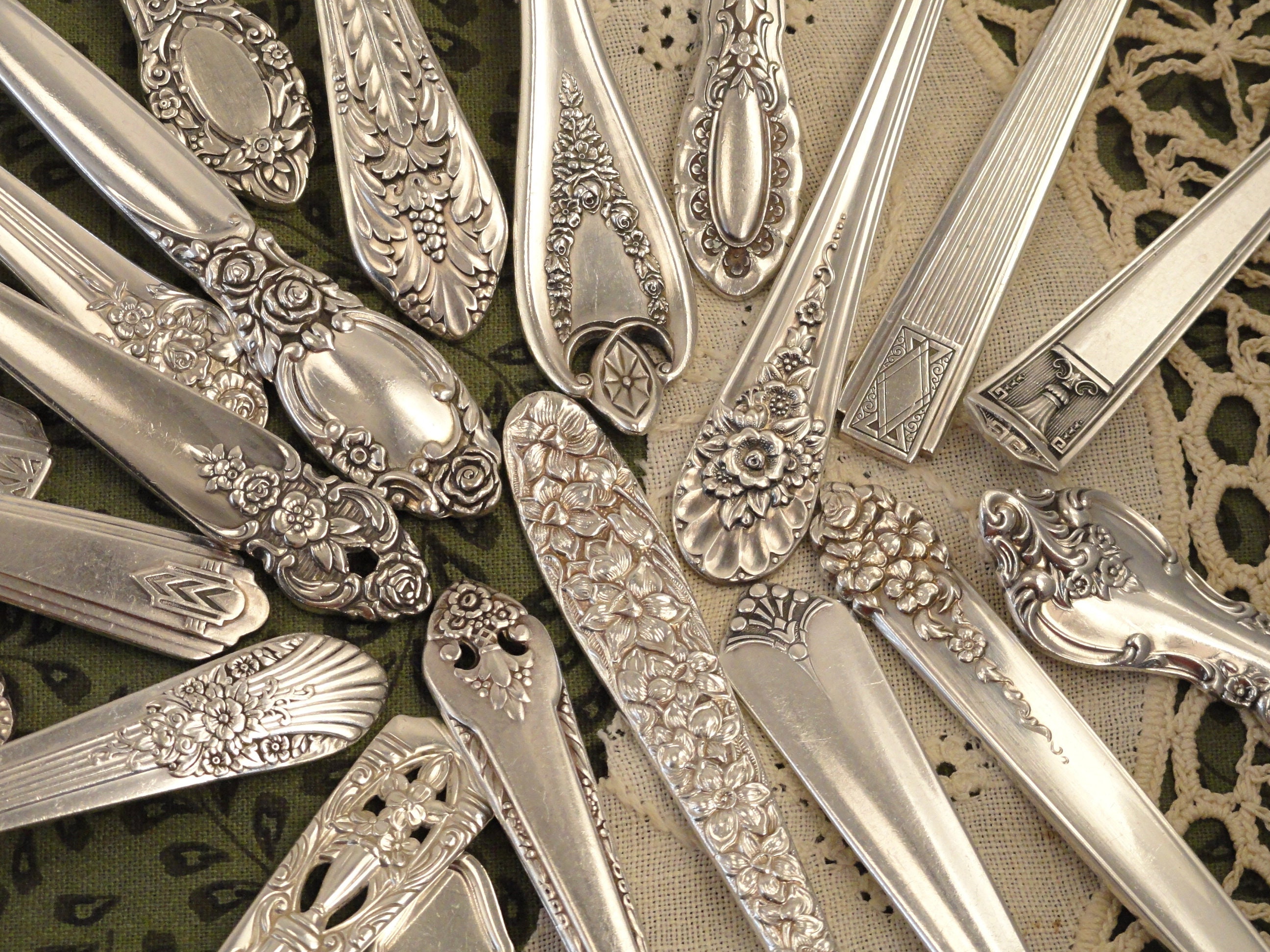The image presents a close-up, color photograph featuring the ornate handles of various pieces of fine silverware, without revealing whether they are forks, knives, or spoons. All of these utensils converge near the center of the frame, displaying about a dozen intricately designed handles. Each handle boasts unique, elaborate patterns including floral motifs, paisley designs, and abstract shapes. Noteworthy features include rose petals, leaf designs, a crest, fan-like embossments, and a diamond pattern, all indicative of hand-embossed craftsmanship, likely in real or sterling silver. The silverware rests on a delicate, white lace tablecloth adorned with green accents, with the tablecloth's intricate lacework especially visible on the right side and center, featuring tightly wound and woven sections with large holes. This setting amplifies the luxurious and detailed nature of the silverware’s ornate designs.